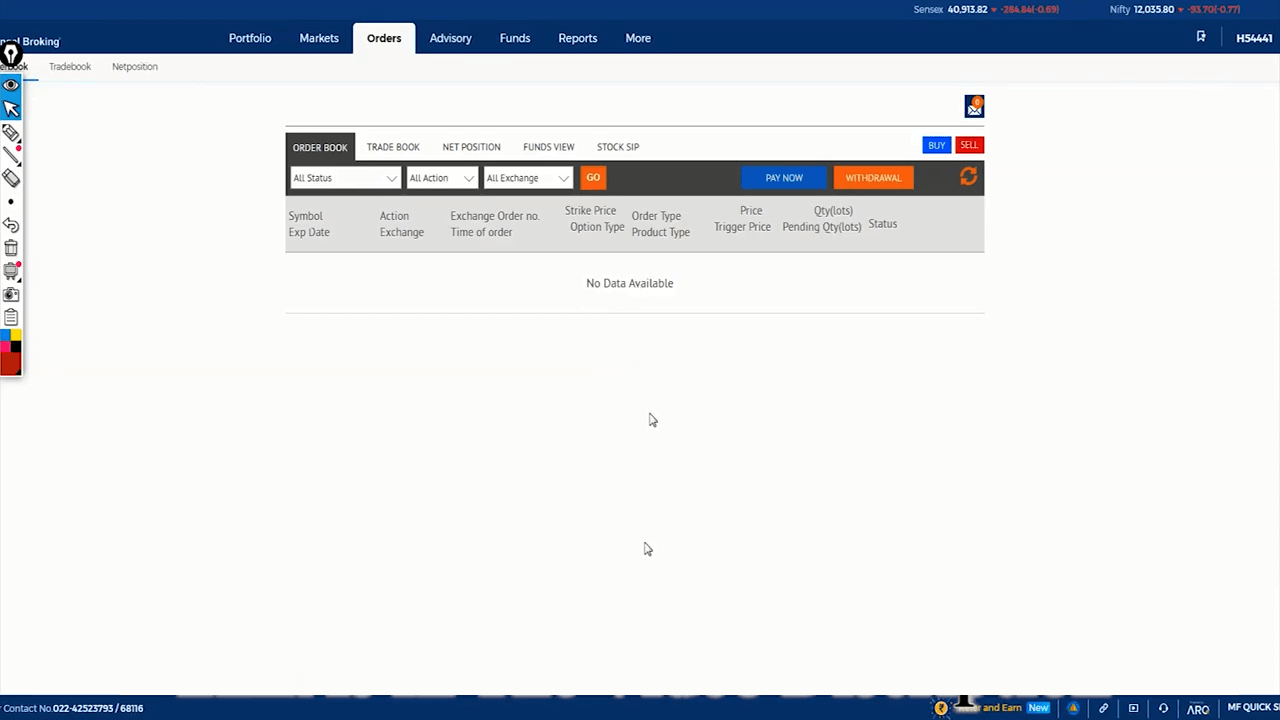This image appears to be a screenshot taken from a computer screen, likely depicting a financial platform interface. The top of the screen features a dark blue navigation bar with several menu options labeled: Portfolio, Markets, Orders, Advisory Funds, Reports, and More. Just below this, the user has selected the "Orders" tab, which is highlighted in a very dark gray color. Within this section, various options are available. 

In the "Orders" section, there are clickable boxes of different colors: some are dark blue, others are orange, and there is a small red box on the far right side. These boxes might represent different actions for managing stock orders. The text throughout the interface is presented in light gray. 

The main background of the screen is predominantly white, creating a clear contrast with the colored interface elements. At the bottom of the screen, there's another dark blue bar resembling a navy blue shade, which contains white text. This lower bar likely serves as an additional navigation or informational footer.